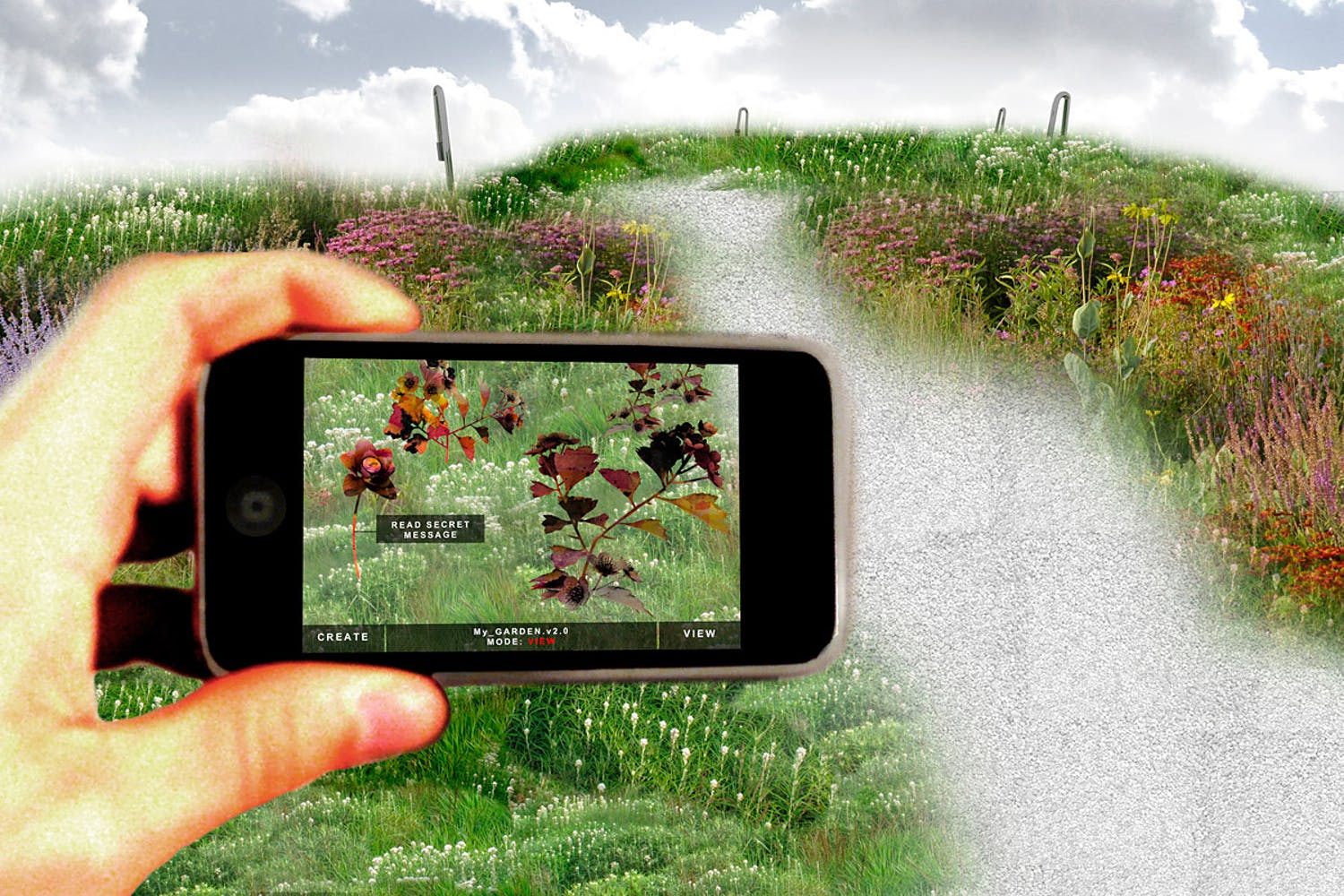The image is a digitally rendered scene depicting a vibrant meadow filled with lush green grass interspersed with orange, yellow, and white flowers. A white gravel path runs through the center of the meadow, flanked by scattered, silver metallic objects that resemble paperclips. The sky above is overcast, featuring a blend of gray and white clouds.

On the left side of the image, a hand is holding up an older model iPhone, capturing a close-up of the flora. The phone screen displays an app interface with various options and the text "Read Sacred Message," suggesting an interactive experience connected to the surrounding environment. The rendering of the elements is somewhat sloppy and blurred, giving the composition an overall artificial appearance. The hand and phone appear to be separately superimposed onto the background of the meadow, adding to the disjointed feel of the image.